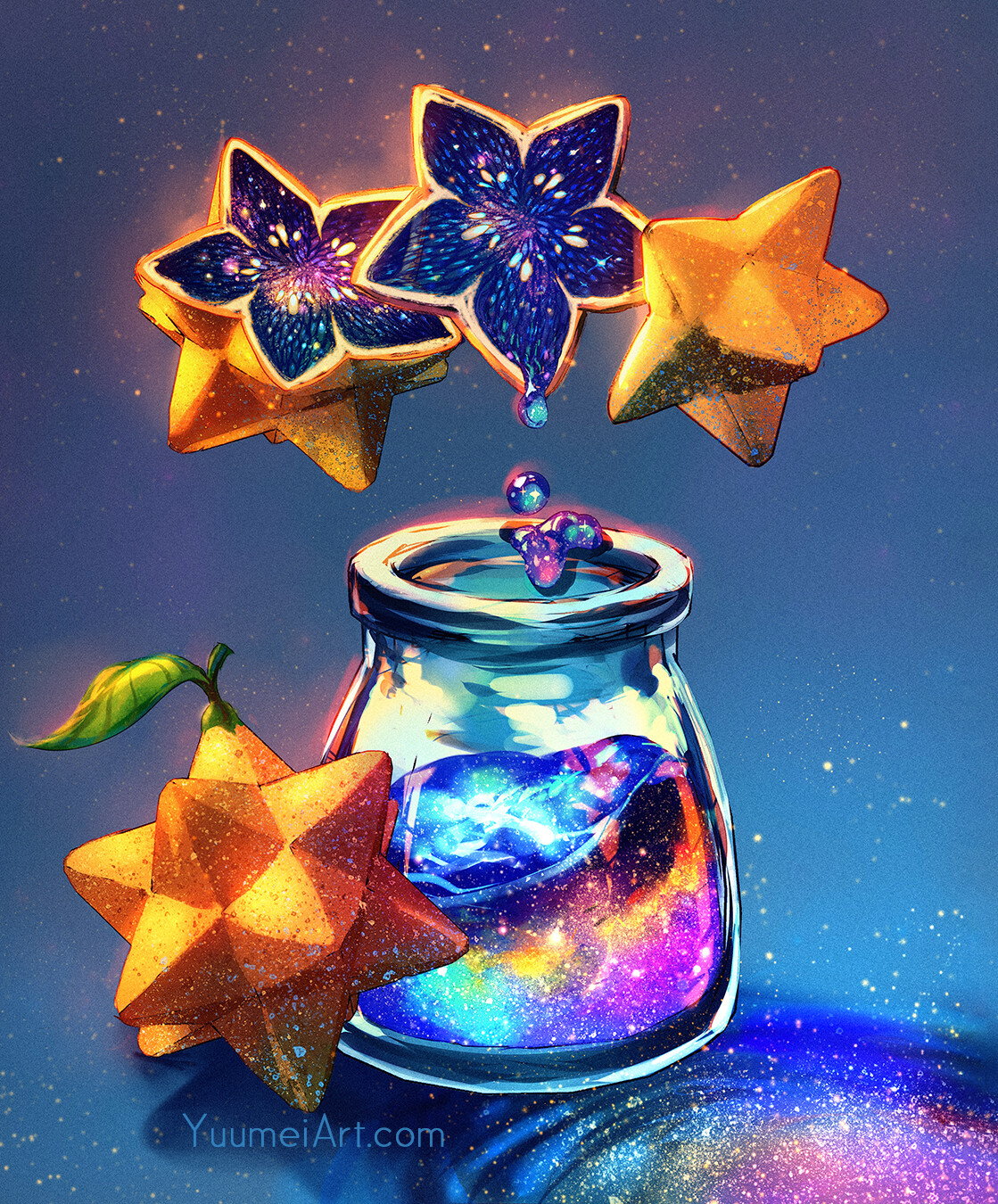The image is a vibrant color illustration, likely created with acrylic paints, set against a gradient blue background that transitions from a lighter blue at the bottom to a darker blue at the top. At the center of the composition is a glass jar resembling an inkwell, filled with a mesmerizing rainbow-colored liquid. Three golden, star-shaped fruits hover above the jar, each intricately sliced open to reveal a blue, pulp-like interior that suggests they are dripping juice or liquid into the jar below.

The fruit, characterized by their unique design reminiscent of Moravian stars, adds an enchanting element to the scene. This becomes more evident as one such star-shaped fruit rests beside the jar on the surface, complete with a stem and leaf, further confirming its fruit identity. The surface beneath the jar reflects the colorful liquid inside, creating an effect similar to a vibrant, miniature galaxy. To the bottom-right corner, a watermark or signature reads "www.yumeiart.com," establishing the artist's identity.

The meticulous details—from the gradient background to the intricate fruit design and the galaxy-like reflections—create an enchanting and surreal visual narrative.